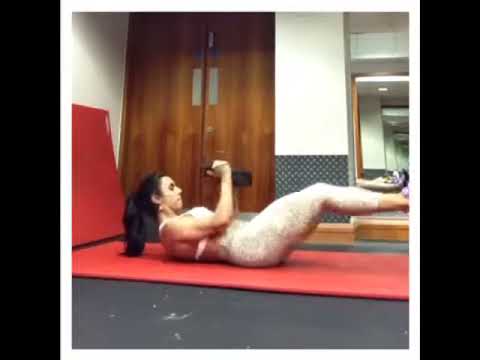The photograph depicts a muscular woman working out in what appears to be a gym or workout room. She is laying on her back on a red exercise mat, positioned towards the bottom of the image, with her legs lifted and her arms tensed as she performs a crunch. She is dressed in white gym attire, including a sports bra and white leggings featuring a grey paisley design. Her dark brown hair is tied back in a ponytail. In the background, the room features double wooden doors with metal push panels located toward the top left, and a mirror on the wall towards the top right where the reflection of her feet can be seen. The setting is indoor, characterized by colors like tan, black, brown, gray, and silver. The entire scene has a slightly blurry quality, adding a dynamic sense of motion to her workout routine.